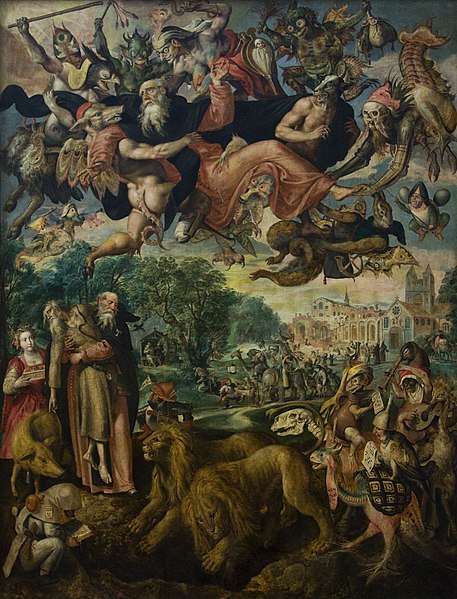This highly detailed and intricate vertical digital artwork resembles an old-style painting and captures a chaotic and fantastical scene. At the center, there is an old man in a robe carrying another old man who appears to be either dead or dying. Surrounding him are various creatures: two lions stand in front, a pig is behind, and there are numerous fantastical beings, including dinosaur-like creatures and a skeleton-headed beast. A woman in a red and gold dress stands in the background near a magnificent castle or large building. The landscape features green trees and a grassy area, contributing to the different tones present in the scene. 

In the upper portion of the artwork, a man looks upward, surrounded by what appear to be pig heads and Egyptian-styled figures. Nearby, there's a pirate-like skeleton fused with a fish, adding to the surreal and bewildering nature of the scene. Throughout the image, the colors used are bold yet muted, ranging from tans and browns at the bottom to more vibrant reds, yellows, greens, and blues in the middle and upper sections. The characters are dressed in old-world style clothing, including long dresses and robes, and the sky is depicted with hues of pinks, blues, and yellows, blending with the myriad of people, demons, and creatures engaged in various activities, including scenes of conflict and despair. Overall, this digital artwork is a mesmerizing confluence of fantastical elements and rich, complex imagery.